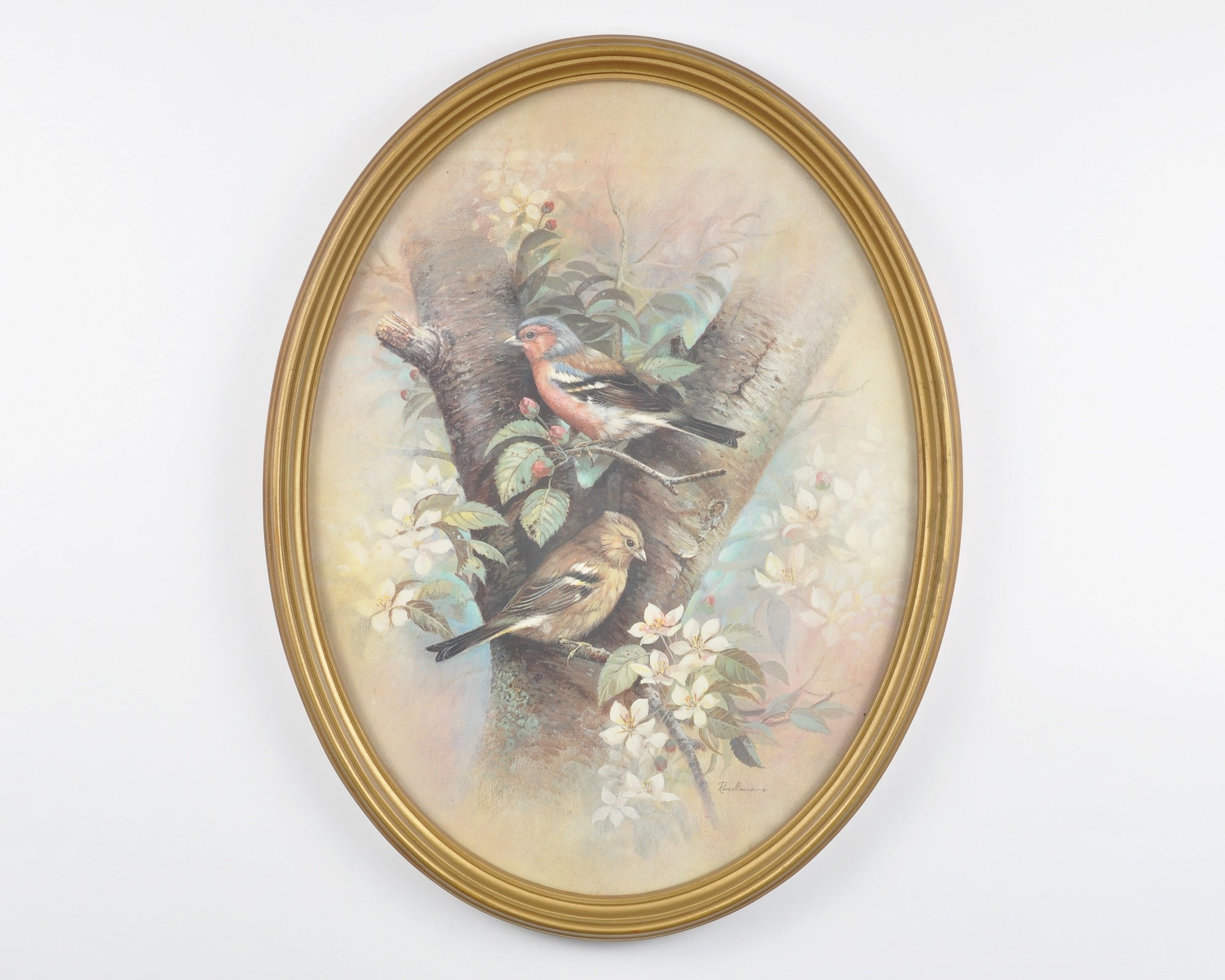This detailed photo captures a piece of home decor featuring a Ruan Manning painting encased in a gold oval frame against a very light gray background. The painting portrays an apple tree that splits into two main branches forming a Y shape. The top branch hosts a reddish-colored bird with hints of blue, which is looking to the left, while the lower branch supports a brown cardinal looking to the right. The tree, adorned with green leaves, white petals, and small red flowers, provides a lively habitat for the birds. The image is artistically faded around the edges, creating an intentional focus on the center scene. A tiny, almost imperceptible signature appears on the bottom right of the painting.